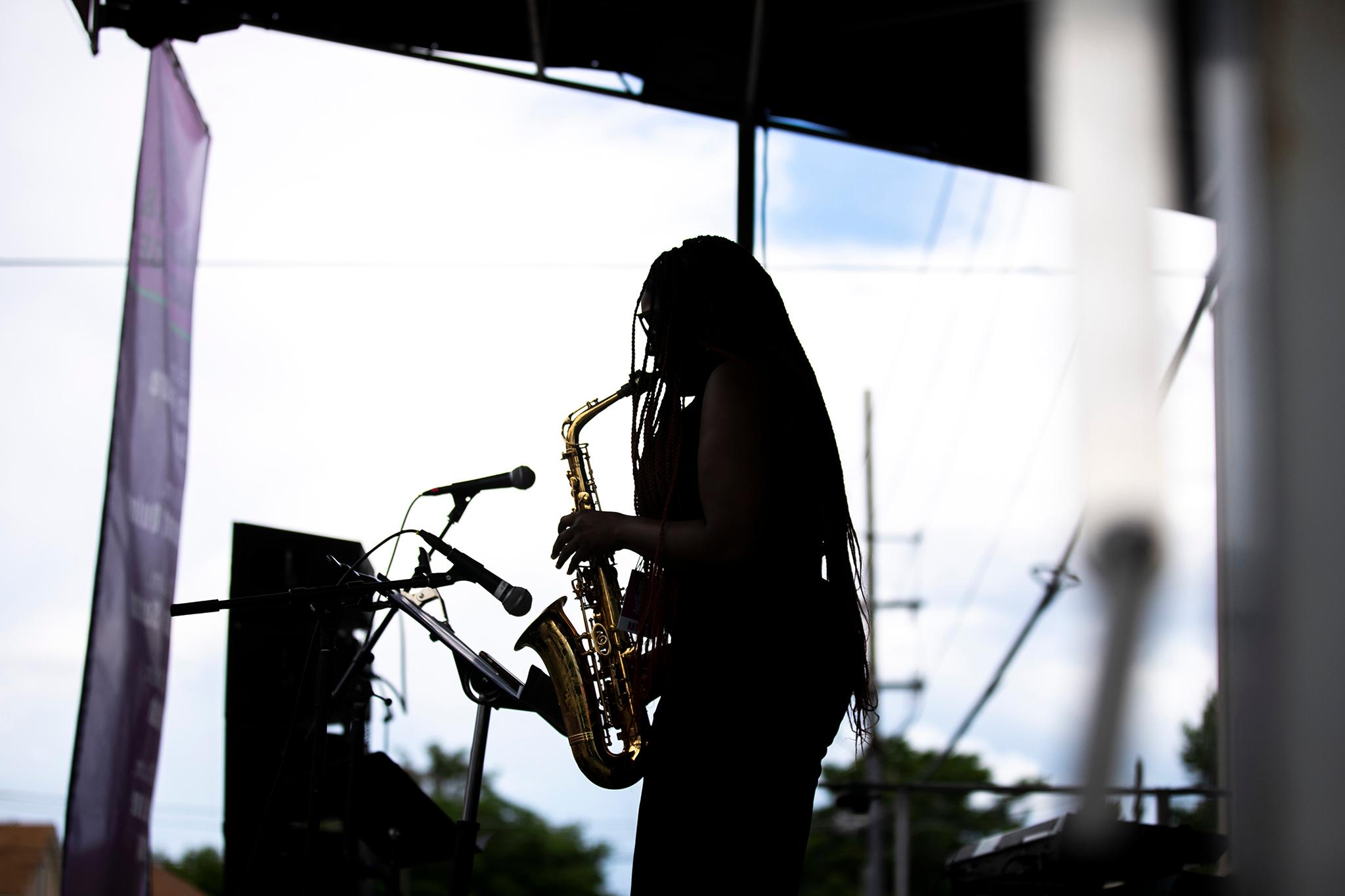The photograph features a silhouetted woman positioned centrally, playing a gold saxophone while standing on a stage. Her side profile reveals long dreadlocked hair and spectacles. She stands in front of two microphones and a rectangular panel, suggesting a live performance setting. The backdrop presents a blue-to-white gradient with the silhouette of trees. Additionally, a huge banner floats from the ceiling on the left, and a dark ceiling projection enhances the ambiance. The scene is further detailed with several pieces of equipment and speakers, accentuating the musical atmosphere.